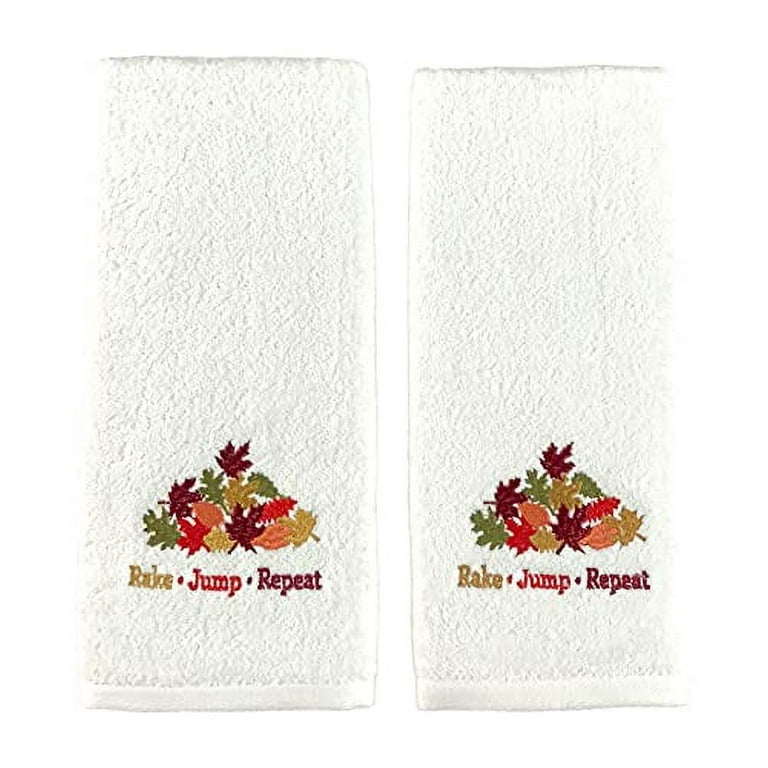This image features two folded white kitchen towels, arranged with their short ends standing upright against a white background. Both towels exhibit a consistent pattern along the bottom edge, which includes an embroidered triangular bouquet of fall leaves in autumnal hues: red, orange, green, yellow, peach, and burgundy. Above this embroidered design, the phrase "rake, jump, repeat" is stitched sequentially in gold, red, and dark red. The towels have a woven texture along the edges and an overall rougher texture, adding to their charming and pleasant aesthetic as part of a fall-themed kitchen decor set.